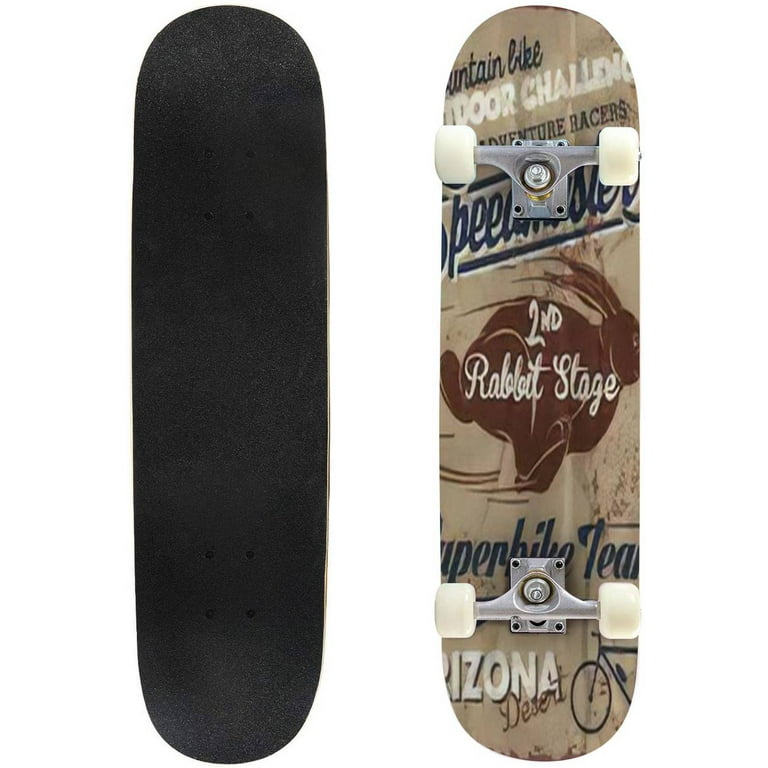The image showcases a skateboard against a completely white background, displaying both its top and bottom views vertically on the screen. The left side of the image illustrates the top of the skateboard, featuring black grip tape and four screws near the top and bottom where the wheels are mounted. The right side reveals the bottom of the skateboard, equipped with white wheels. Dominating the center of the deck is a large burgundy rabbit, seemingly hopping towards the right, with the words "Second Rabbit Stage" inscribed in white across its body. The deck also bears various inscriptions: "Mountain Bike" in dark blue at the top, followed by "Outdoor Challenge" in white, "Adventure Racers" in black, and cursive writing partially obscured by the wheels, stating something akin to "Super Bike Team." The design extends across the deck, capturing a sense of adventurous spirit, reminiscent of the Arizona desert with an additional graphic of a red rabbit and partial bicycle.